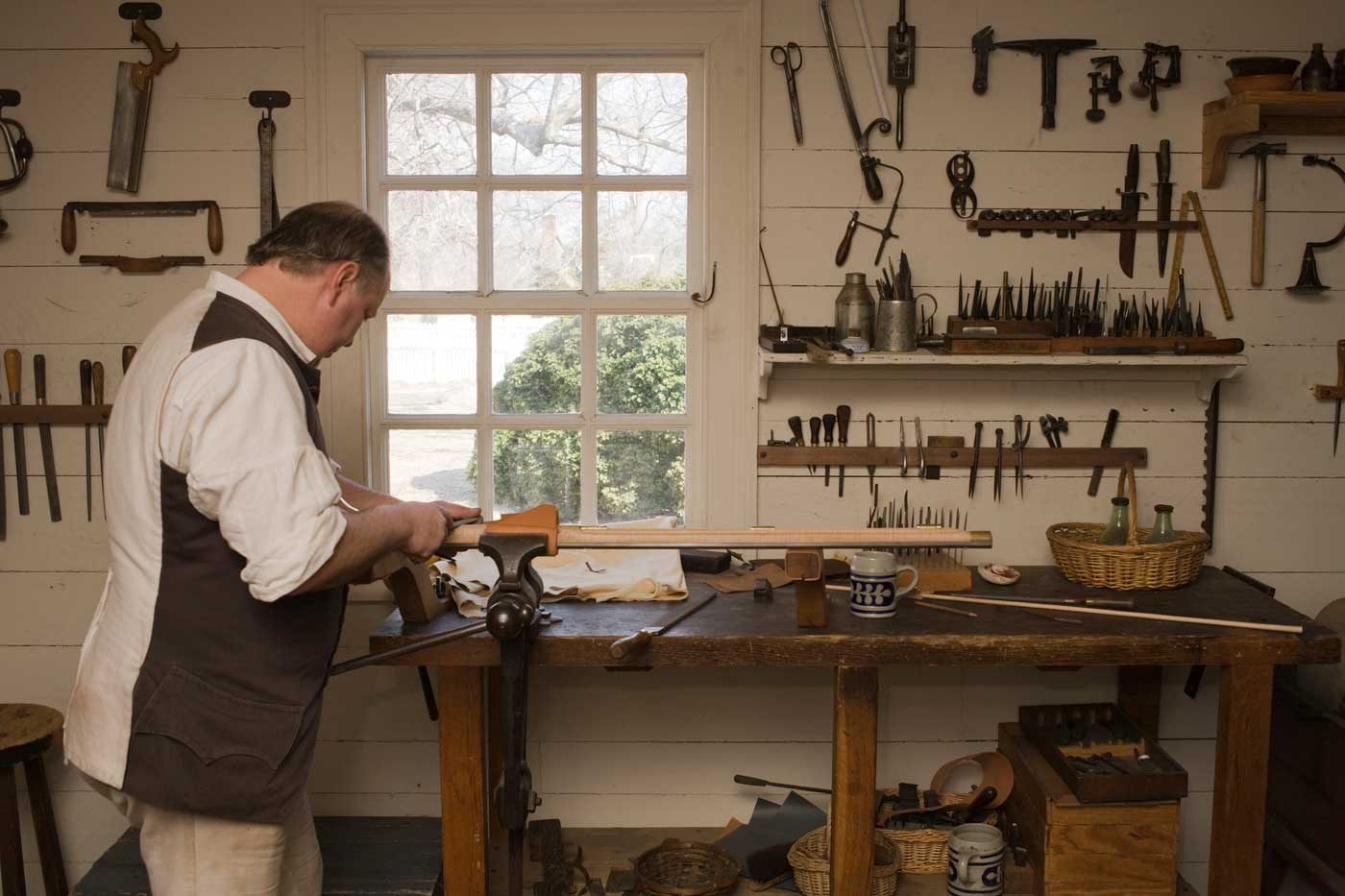In this photograph, a man is intensely focused on woodworking at an old-fashioned wooden tool bench within what appears to be his garage workshop. He is skillfully shaving down a brown rod clamped to the table with a knife. He is dressed in khaki pants and a layered outfit of a brown and white vest over a white long-sleeved shirt with sleeves rolled up to his elbows. His gray hair is slightly balding at the top. The tool bench is surrounded by shelves and racks holding a wide variety of hand tools, including picks, needles, carvers, saws, scissors, hammers, and rulers, indicating his advanced carpentry skills. 

Behind him, the white paneled wall is adorned with numerous hanging tools, while a window with a grid of four rows of three squares frames a bright day outside, showcasing bare trees and shrubs suggesting a fall setting. Below the workbench, there is a coffee mug with a blue pattern, accompanied by baskets and boxes, adding a touch of personal clutter to the organized workspace.